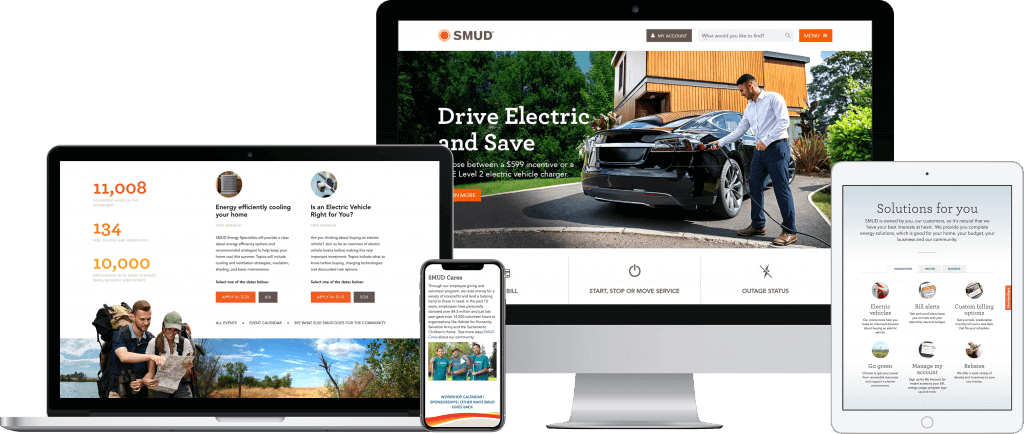**Detailed Caption:**

The image showcases a variety of screens, all seemingly related to electric vehicles and energy solutions, against a multitiered backdrop. 

1. **Background Computer Monitor**: 
   - Positioned in the background, the computer monitor displays a man plugging a wire into his electric car.
   - To his left, the text reads "Drive Electric and Save" in white lettering.
   - Above the screen is a white banner with the letters "SMUD" next to an orange symbol.
   - At the bottom of the monitor, there is another white banner displaying additional options in dark gray lettering.
   - The monitor has a silver edge at the bottom and sits on a silver stand.

2. **Left Tablet Screen**: 
   - On the far left, there is a large tablet or iPad displaying a partially white background with orange and yellow lettering.
   - Detailed dark black letters further explain the content.
   - The bottom of the screen depicts a picturesque wilderness scene, transitioning from grasslands and woodlands to a distant lake or ocean.
   - Foreground includes a man and a woman with backpacks, holding a map. The woman wears a cap.

3. **Middle Smartphone Screen**: 
   - To the right of the tablet, a vertically oriented smartphone displays the text "SMUD Cares" in black font at the top.
   - Below this headline, there is an image of three men wearing turquoise t-shirts.
   - Further down, blue lettering is visible along with a curved design featuring orange and gray artwork.

4. **Right Tablet Screen**: 
   - Positioned on the far right, a smaller tablet, roughly Kindle-sized, has a white background.
   - The center of the screen features a blue and white themed rectangle with the words "Solutions for You" at the top.
   - Below this, there are six informational icons, each inside round circles with text underneath in dark font.
   - An orange vertically oriented rectangle with white font occupies the extreme right edge of the screen.

Each device displays content that conveys information about electric vehicles, energy-saving tips, and related services provided by SMUD.